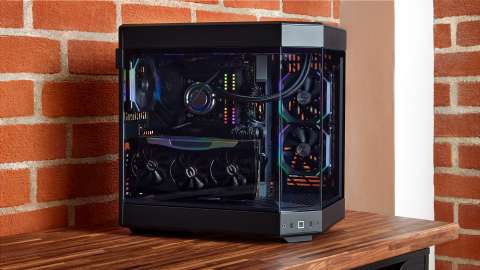The photograph features a central black electronic device, which resembles a gaming PC tower. The device has a black top and bottom, with its middle section composed of translucent material, allowing a view of its internal components, including wires, fans, and other electronic parts. Subtle rainbow-colored lighting adds a dynamic effect to the internals. The tower is situated on a wooden counter, showcasing a pattern of alternating light and dark wood stripes. To the left of the device is a uniformly colored brick wall with whitish-gray grout, and behind it, a white beam is visible against another brick wall. This setting harmoniously combines the textured complexity of the device with the rustic elements of the wooden counter and brick walls.